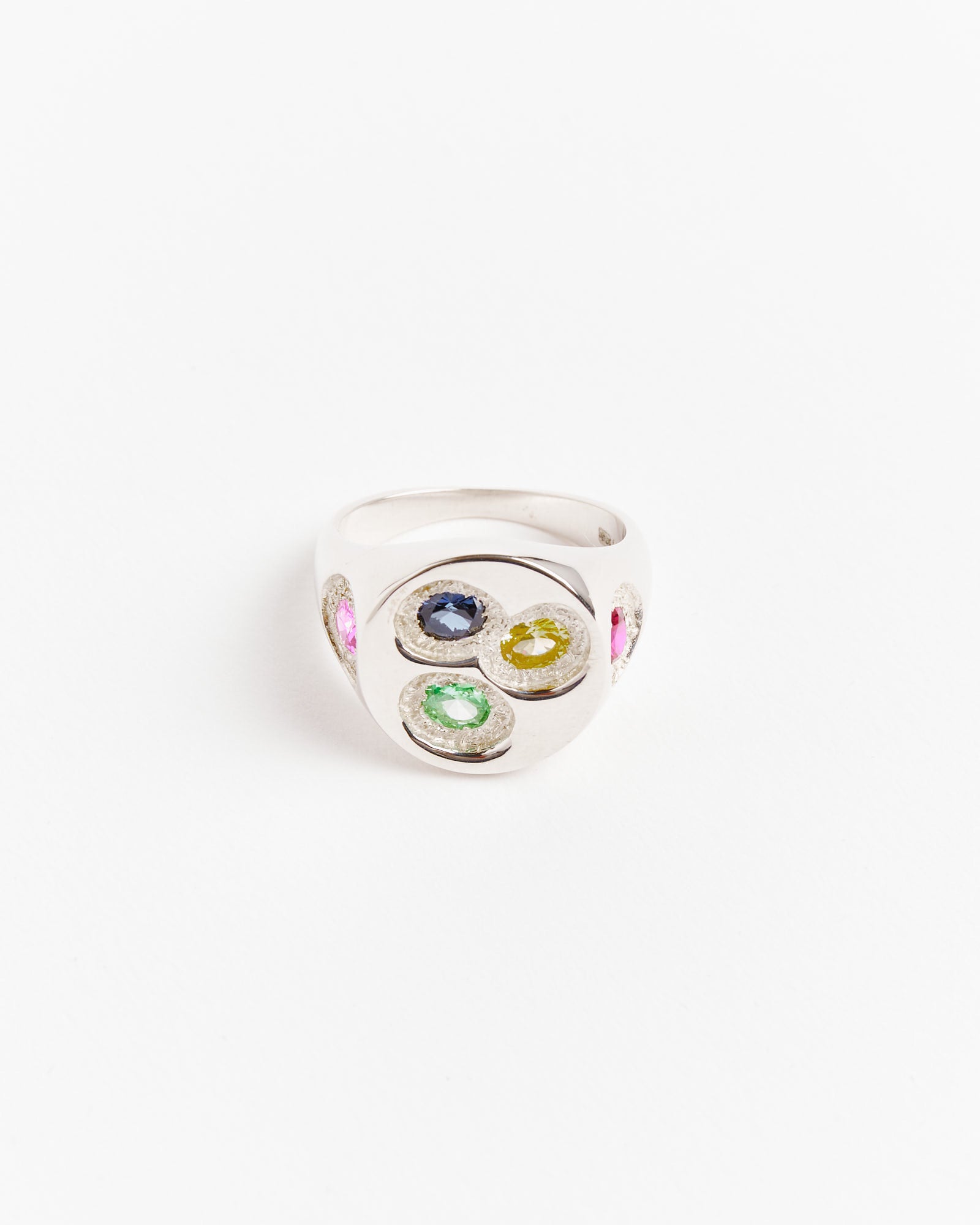The image features a highly reflective, metallic ring, likely made of silver or a similar white metal such as platinum or chrome, placed centrally within a white photo box. The ring's top surface showcases three prominent gemstones: a vivid blue sapphire, a bright yellow citrine, and an eye-catching green emerald, each encircled by what appear to be diamonds or simulated diamond accents. Flanking these central stones on either side of the band are two additional gemstones, distinguished by their pink hue and also bordered by diamond-like stones. The reflective quality of the ring's metal mirrors the white surroundings, enhancing its sleek, shiny appearance. The careful arrangement of the ring and the light source coming from the right of the image accentuate the vibrant colors of the gemstones and the sparkling diamond borders.